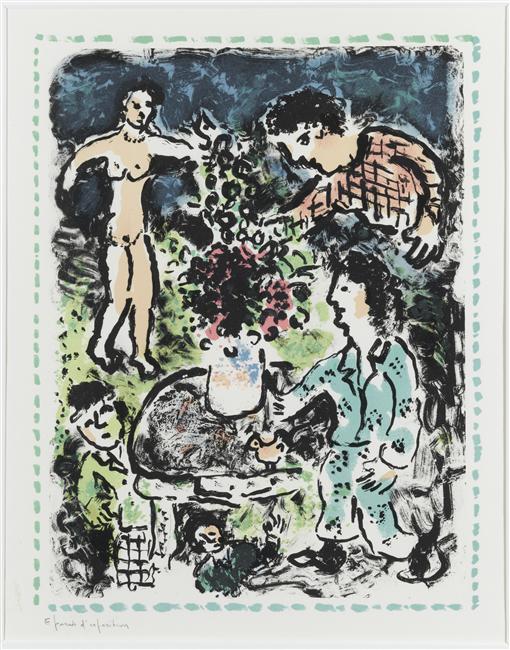The drawing, rendered in a Matisse-like watercolor style, captures the chaotic morning scene of a typical household. Central to the composition is a gray table set on a green, grassy background. A white vase brimming with vibrant orange, pink, and green flowers sits atop the table. Surrounding the table are three children in various states of morning disarray: one child with dark hair, checkered pants, and a gray blouse hides beneath the table; another child stands next to it, while a third child seems poised to push the vase off the table.

A harried father, dressed in a pink checkered shirt, leans over the table, seemingly struggling to restore order. To the right of the table, a woman with long black hair sits calmly in a coral-colored outfit, appearing to be a stabilizing presence amidst the chaos. In a striking and somewhat surreal detail, the upper left of the image features a depiction of another woman, this one naked, standing with her hand extended, an enigmatic figure perhaps symbolizing the mother's overwhelmed state as she enters the room.

The entire scene is enclosed within a frame of discontinuous dotted lines, adding to the sense of frenetic energy. The background transitions from a dark gray at the top to a green grassy area where the table and figures reside, infusing the scene with a blend of domesticity and artistic abstraction.